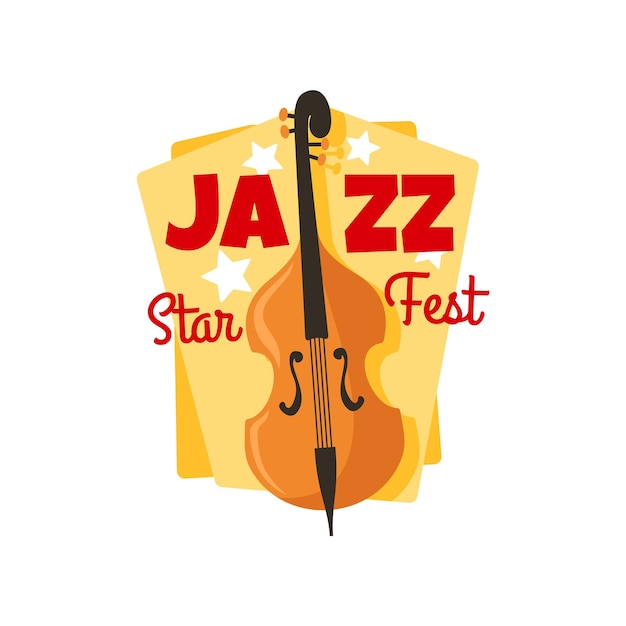The image features a traditional-styled, animated violin with a medium brown to deep orange wooden hue. The violin is positioned at the center of the image, effectively separating the words. The violin has black strings and middle pieces, adding to its detailed depiction. Surrounding the violin, the background incorporates a unique geometric design resembling overlapping coffin shapes—one in mustard yellow and the other in light yellow—to create depth. Boldly displayed across the violin are the words "JAZZ STARFEST" in red letters; "JAZZ" is capitalized, large, and bold, while "STARFEST" is written in a thinner cursive style. Additionally, four white stars adorn the background, enhancing the visual appeal. The violin casts a shadow that matches the yellow background overlay, emphasizing the three-dimensional effect.